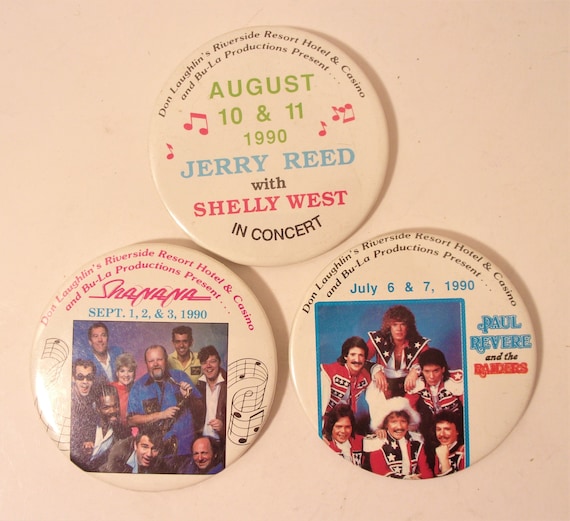The image features three white, circular concert buttons displayed against a light beige background, arranged in a triangular formation with one at the top and two below. Each button measures the same size. 

The top button highlights a Jerry Reed with Shelly West concert, dated August 10 and 11, 1990. This button features green and blue text detailing the event.

The bottom-left button promotes a Sha Na Na concert, which is co-organized by Don Laughlin's Riverside Resort, Hotel, and Casino, and Bula Productions. It features pink text with musical notes surrounding a photograph of the nine-member band and is dated September 1, 2, and 3, 1990.

The bottom-right button advertises a concert by Paul Revere and the Raiders, also organized by Don Laughlin's Riverside Resort, Hotel, and Casino, and Bula Productions. Dated July 6 and 7, 1990, it includes a photograph of the band in their red, white, and blue outfits and features blue, black, and red text.